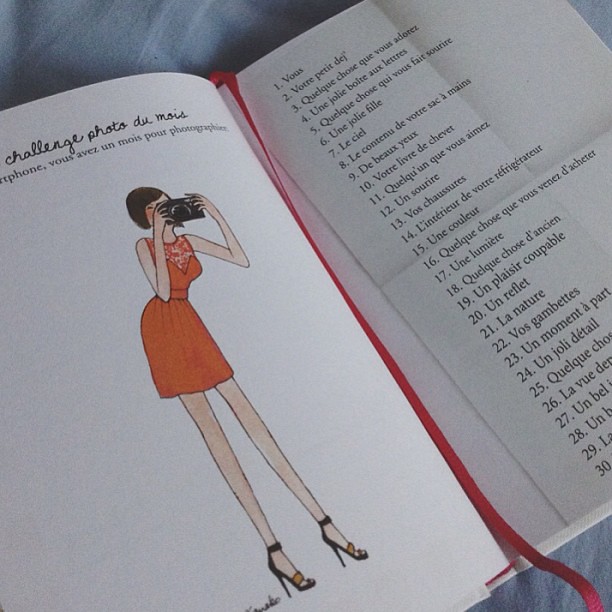The image depicts an open book, presumably a French textbook, featuring a left-hand page with an illustration and a right-hand page with text. The left page showcases a woman with long legs and black high heels, pointing straight down. She is dressed in an orange dress with a flowery pattern at the top around her shoulders and chest. The woman, who has short hair at chin length and fair skin, holds a camera up to her face as if taking a photo. Above her, in cursive, is the text "Challenge Photo du Moi," and below that, in French, it states, "Vous avez un mois pour photographier." 

On the right-hand page, a piece of paper partially covers it, but a numbered list from 1 to 30 is visible, featuring various French phrases starting with "Vous" and "Votre petit." The writing is in black ink. A red ribbon bookmark runs vertically down the center of the book, trailing to the bottom right corner, indicating a placeholder. This detailed setup suggests it is an instructional page, likely aiding in vocabulary or phrase memorization.